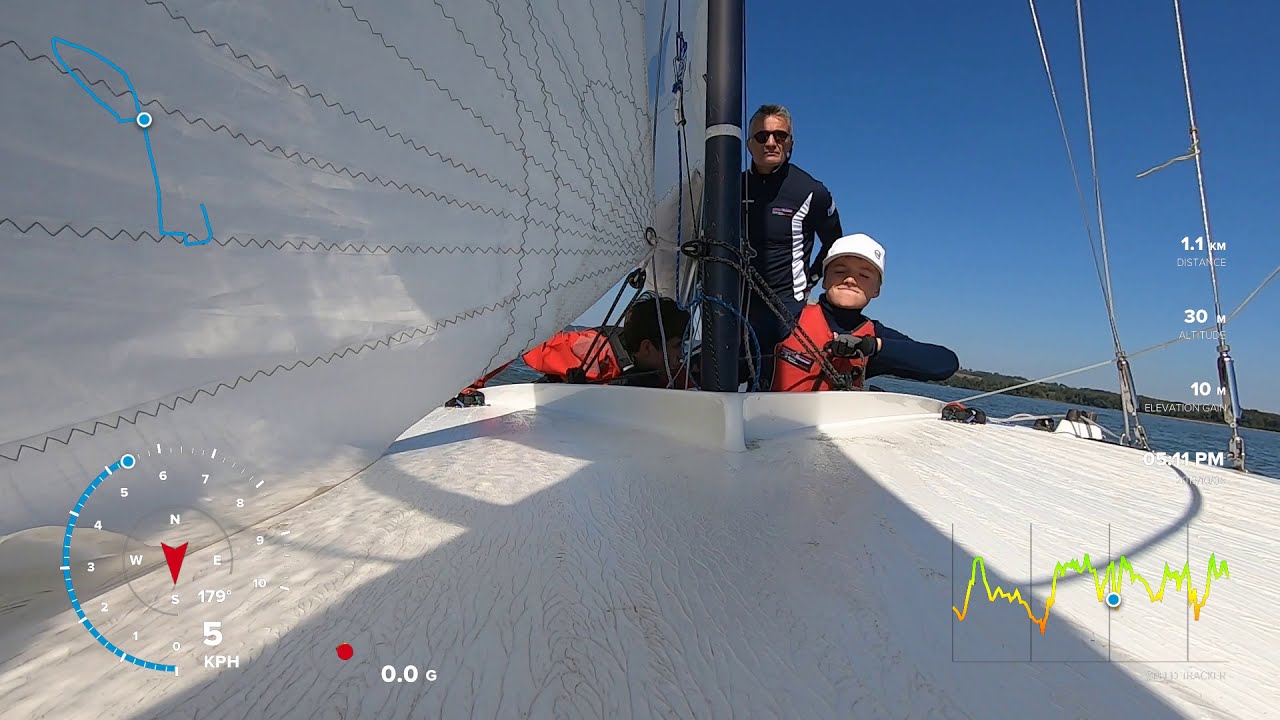In this vibrant outdoor photograph, taken on a brightly lit, clear blue-skied day, a man, a young boy, and a woman are seen aboard a sailboat against a backdrop of shimmering water and a forested shoreline. The sailboat itself is white, with a large, striking white sail extending upward from a central black mast. The main focus is on the man and the young boy, likely around eight or ten years old, who appears to be his son. The man, positioned behind the mast, is dressed in a black and white striped long-sleeved shirt and sunglasses, exuding a confident stance as he looks directly ahead. The boy, in front of him, is engaged with the ropes, wearing an orange life jacket, a black shirt, and a white baseball cap, his face showing a playful smirk with eyes closed as he strains to manage the sail. To their left, a woman—possibly the boy's mother—is also seen, assisting the boy with the sail, donning a life jacket as well. Together, they create a dynamic scene of family teamwork and enjoyment on the calm, picturesque waters.